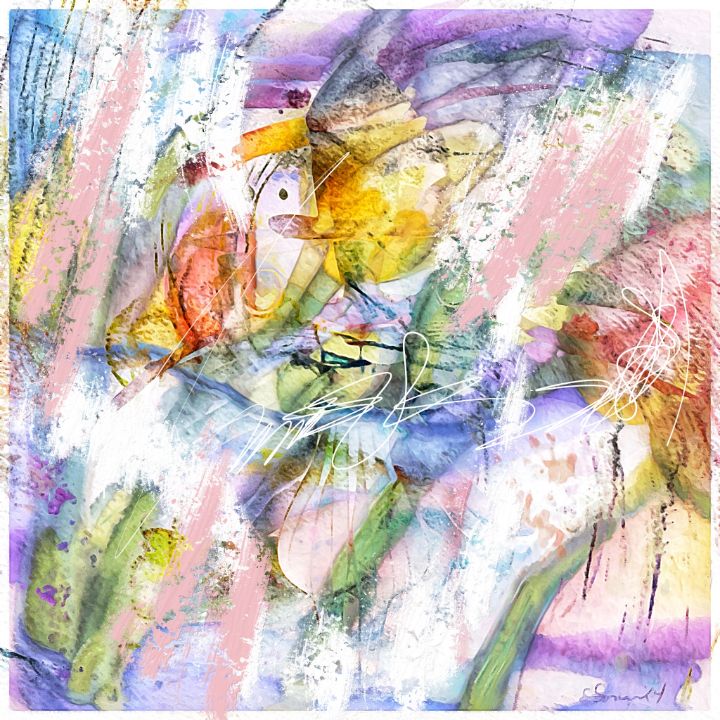This image showcases an abstract watercolor painting characterized by a kaleidoscope of vibrant colors, including yellow, white, purple, blue, light blue, lime green, dark blue, pink, beige, and darker yellow. The entire image is densely packed with splashes and elongated brushstrokes of color, creating a lively and dynamic composition. The painting features a predominantly purple section in the upper center that transitions into yellow and green, with hints of red. Towards the upper left, blue merges into pink, while the right-hand side of the painting presents red and yellow resembling a flower stalk fading into green. The bottom right area is dominated by purples with additional shades of blue and green. Hidden within the tumultuous array of colors, there also appears to be an ink outline resembling a shark with its head up and mouth open. The artist has signed their name in white near the center of the piece, adding a personal touch to the nearly entirely colored canvas with just a minimal presence of white background. The painting is highly abstract, with no clear depiction of plants or animals, and could easily be envisioned hanging in a modern art museum.